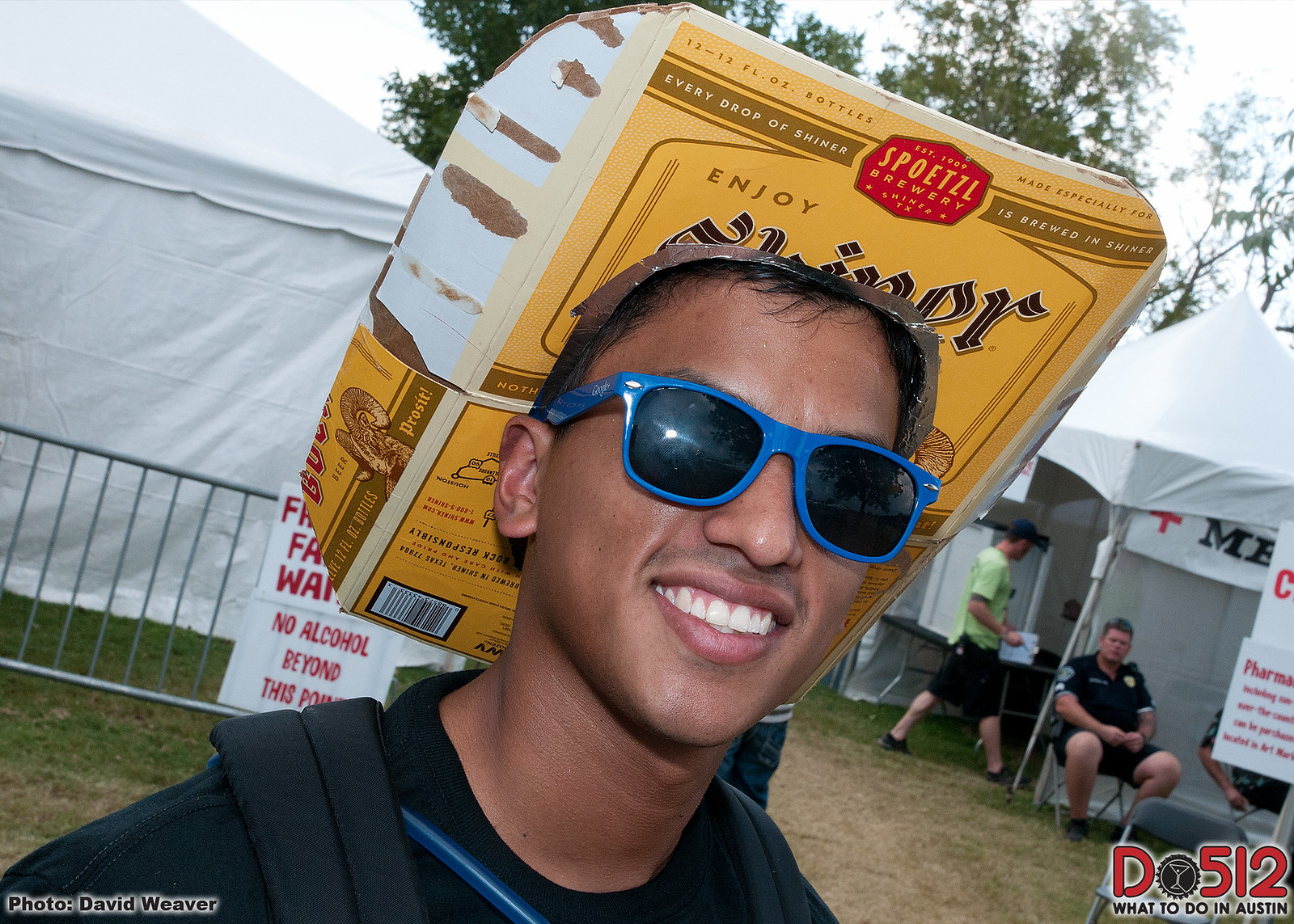In this close-up daytime photograph taken at an outdoor event or festival in Austin, a man of likely Puerto Rican or Mexican descent stands smiling at the camera. He sports a unique, makeshift hat crafted from a Scheinerbach beer cardboard case and wears blue sunglasses with black frames. His short black hair complements his darker skin tone, and a black polo shirt with blue accents along with a black backpack with visible straps completes his attire. 

The background reveals a bustling festival atmosphere, with a white canopy tent and a metal fence with vertical poles. To the right, a police officer in a black uniform sits on a chair, adding to the sense of a monitored event. Text in the bottom right corner reads "Do 512" alongside a martini glass logo, accompanied by the tagline, "What to do in Austin," and a photographer credit to David Weaver in the lower left. The light sky above and various attendees moving past, including someone in a green shirt and black shorts, further set the scene.